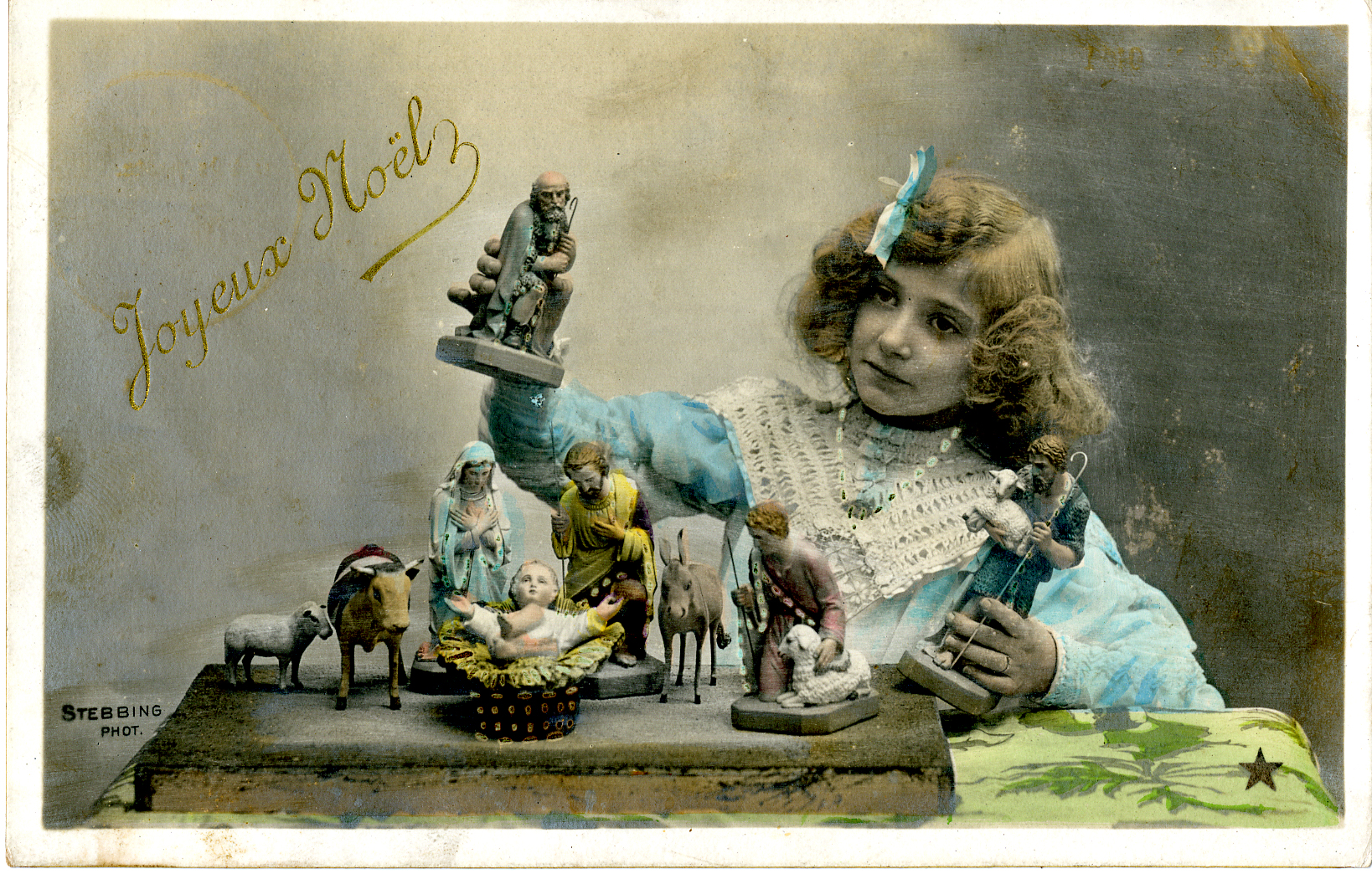This old, colorized antique postcard from the early 1900s depicts a young girl, likely aged around 12 to 14, standing in front of a display of nativity figurines. Her hair, styled in short, crimped curls with a blue bow, complements her Victorian-style light blue dress adorned with lace. She also wears a pearl necklace. The girl's hands hold two figurines; one is a shepherd, and the other may be a figure holding a lamb. The table before her features a detailed array of nativity figures, including the baby Jesus in a manger, Mary, Joseph, various shepherds, wise men, sheep, a donkey, and an ox. The image, initially black and white and later colorized, is bordered in white with gold diagonal lettering at the top left reading "Joyeux Noel." The artist's name, Stebbing Vogt, is inscribed at the bottom left. The colors and toning of the image reflect vintage photographic colorization techniques.